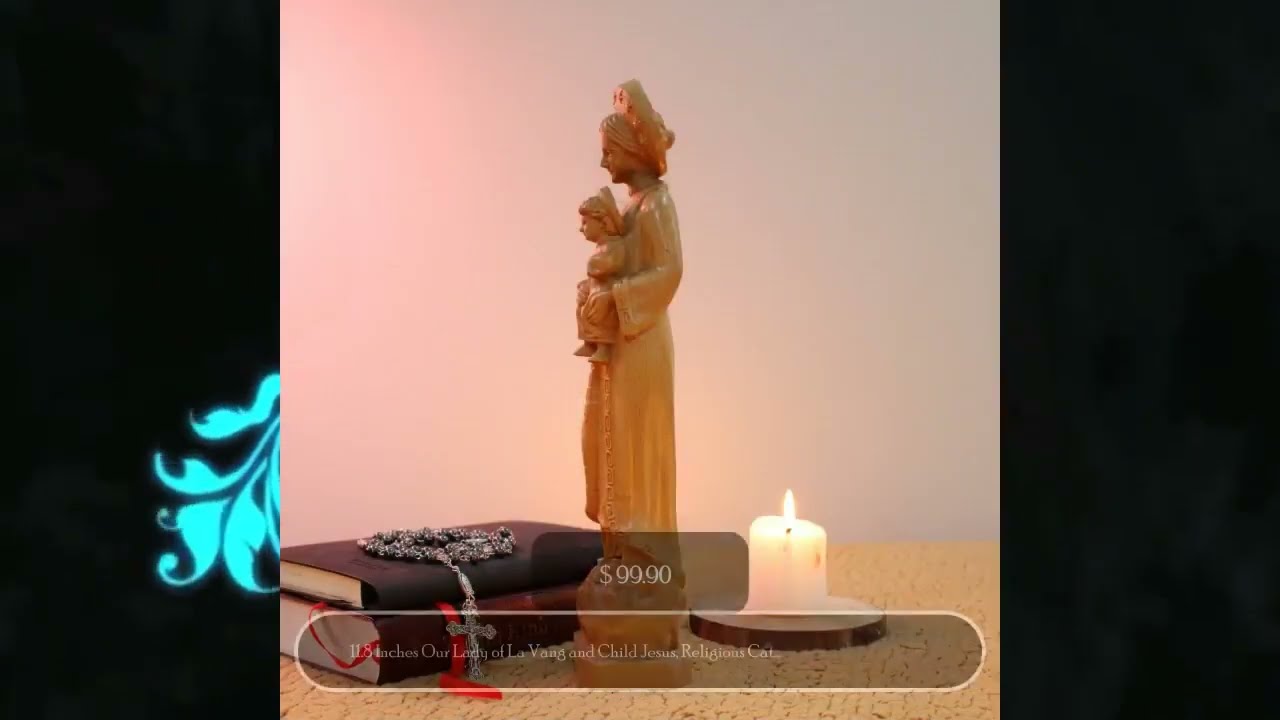This image depicts a promotional setup for what appears to be a religious item for sale, possibly from a shopping channel or an advertisement. Central to the image is a detailed statue of "Our Lady of La Vang" holding the Child Jesus, both depicted with straight postures. The statue has a creamy caramel color and features a halo-like round piece on the woman's head. She is clad in a long robe and stands on a stone base. To the right of the statue is a lit white candle on a round coaster, while to the left are two books, one resembling a Bible, with a rosary draped over them and its steel cross discernible. 

The scene is set against a textured beige tabletop with a gradient background that shifts from pinkish on the left to blue on the right. The image is framed with a thick border, variegated in gray and black with touches of bright blue on the left side. An overlay indicates the price of the statue, listed as $99.90, along with text at the bottom that is difficult to read but mentions "11.8 inches, Our Lady of La Vang and Child Jesus," suggesting the statue's dimensions and subject.